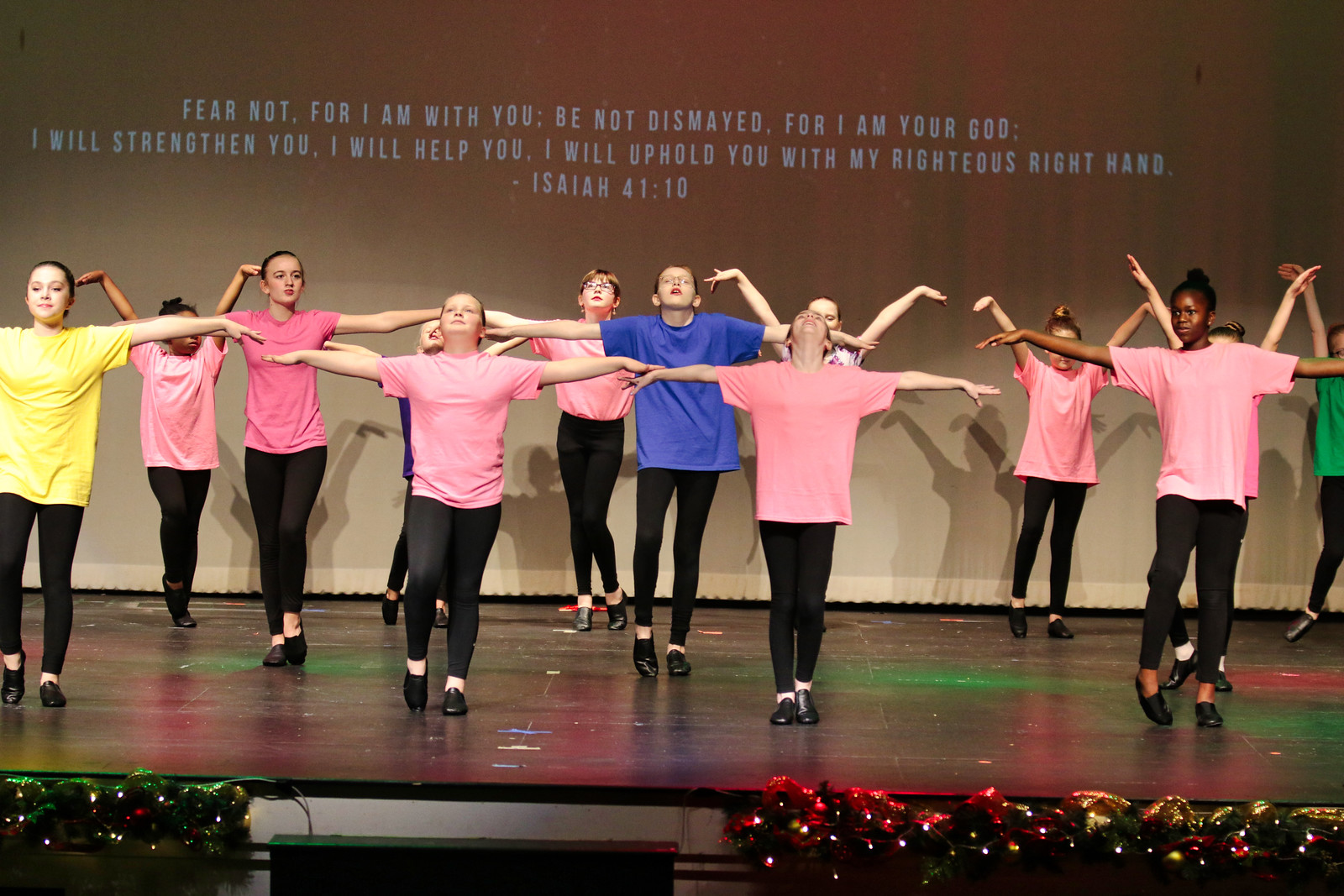This color photograph captures a lively stage performance by approximately fourteen children, seemingly engaging in a coordinated singing and dancing presentation. The performers, arranged in three rows, have their arms outstretched, striking a pose in unison. They are all dressed in black pants and black shoes, adorned with pastel-colored t-shirts in a variety of shades: predominantly pink, with notable exceptions including one child in a blue shirt at the center, another in a yellow shirt on the far left, and one more in green at the back right corner. The stage is decorated festively with Christmas lights, decorations, and greenery, creating a joyful ambiance. A large white curtain serves as the backdrop, onto which a Bible verse from Isaiah 41:10 is projected, reading: "Fear not, for I am with you; be not dismayed, for I am your God. I will strengthen you, I will help you, I will uphold you with my righteous right hand." Red and green spotlights illuminate the floor of the stage, adding a vibrant touch to the scene.